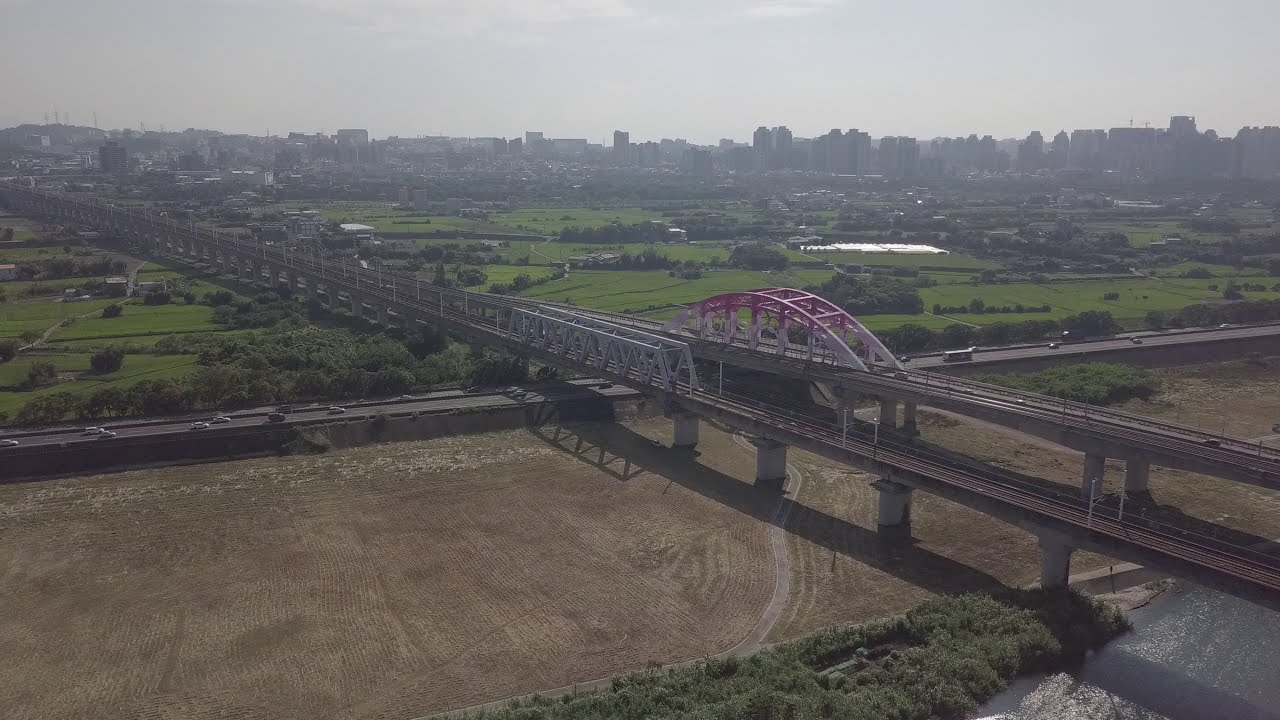The image captures a high-angle, drone-shot view of an extensive bridge and road network over a varied landscape. Dominating the scene is a two-level train bridge with a distinct red and white arch, stretching diagonally from the bottom right to the top left of the image. This bridge crosses a combination of terrain, from a dry riverbed—maintained and mowed, resembling farmland—to a smooth, flat dirt area and patches of water. Parallel to the train bridge is another elevated structure, a four-lane highway bustling with heavy traffic. The bridges sit on concrete stilts, with the highway running underneath them. Beyond these structures, the landscape transitions into grassy fields, small lakes, and scattered woodlands. In the hazy, smoggy distance, a city skyline with towering high-rises and industrial elements can be seen, suggesting a northeastern urban environment, akin to Pittsburgh. The scene is shrouded in a bright yet cloudy, gray sky, enhancing the industrial and sprawling nature of the setting.